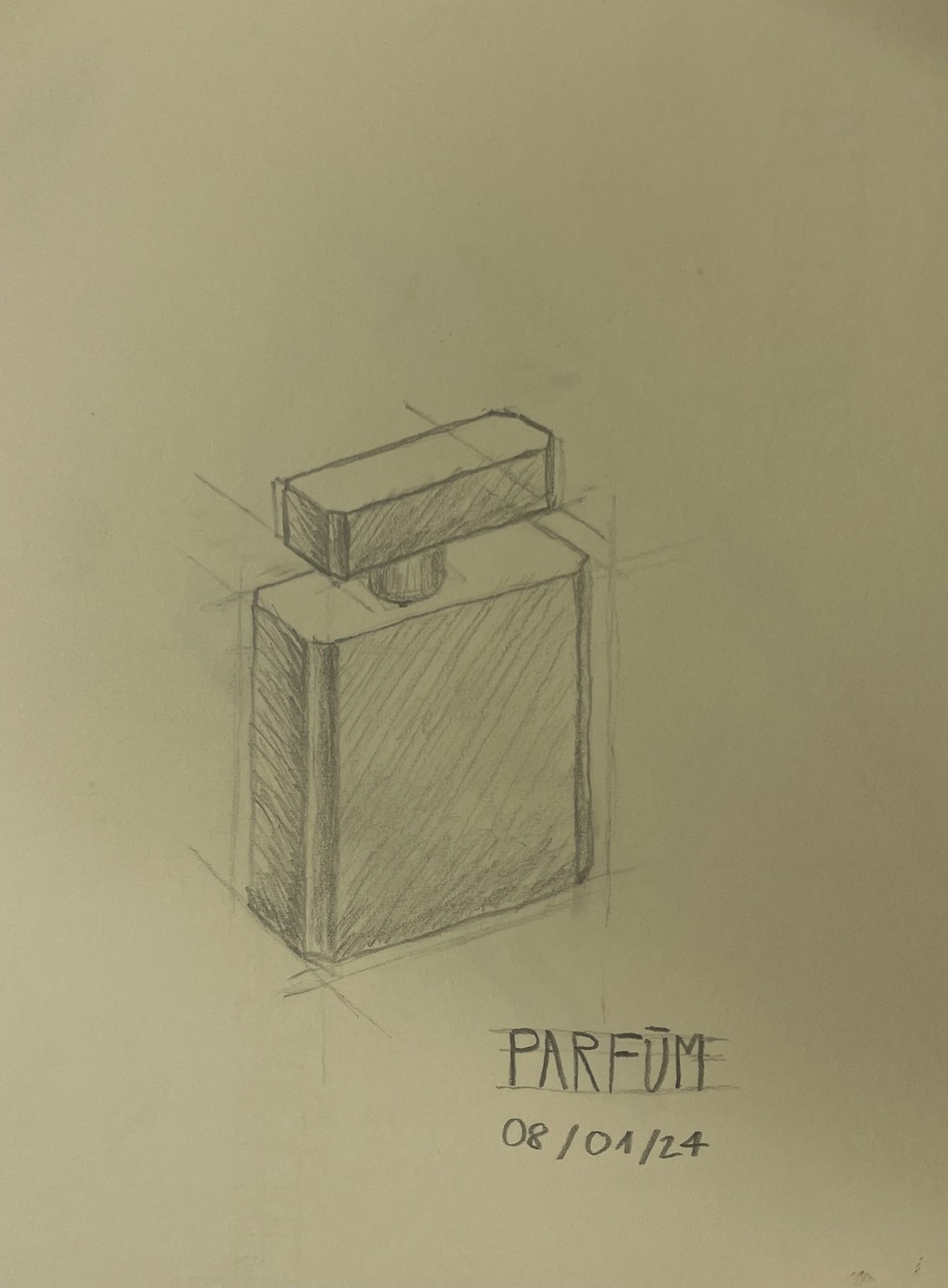The photograph captures a hand-drawn image of a simple, unadorned perfume bottle, sketched with a pencil on white paper. The drawing clearly shows the bottle's contours, with visible individual pencil lines adding texture and dimension through techniques such as diagonal shading. The bottom of the drawing features the word "Parfum," spelled P-A-R-F-U-M, potentially with an accent mark over the 'U'. Below this, the date "08/04/24" is penned, indicating either April 8th, 2024, or August 4th, 2024, depending on the date format used. The paper itself bears slight pencil smudges and minor wrinkling. The overall aesthetic is monochromatic, utilizing shades of gray against the white paper background.